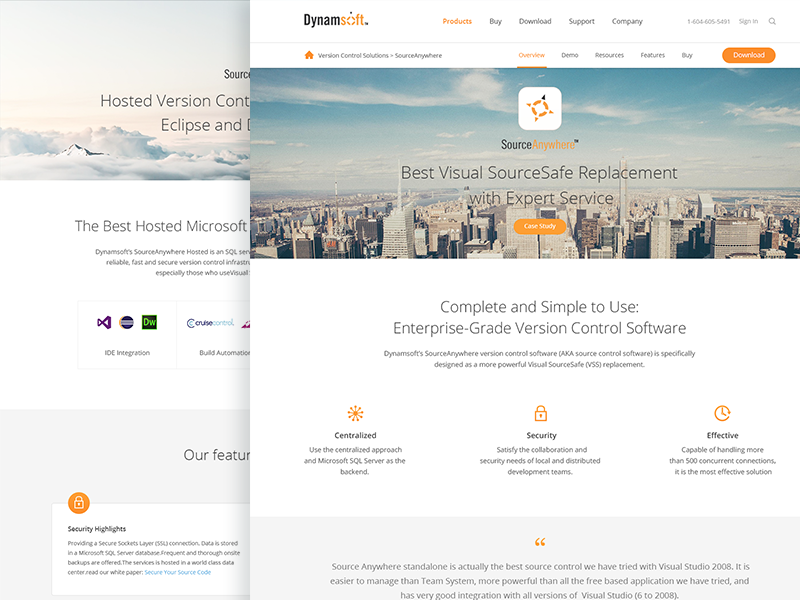The image frame is a slightly horizontal rectangle containing two screen grabs likely from the same website. The left image is a vertically rectangular fragment displaying partial text. Key visible phrases include "hosted version," "Eclipse," "the best hosted Microsoft," "our features," and "security highlights." 

Adjacent to this, on the right, is a fuller view of the Dynamsoft website, although its left edge appears cropped. At the top of this image, the Dynamsoft logo is visible along with menu headings for pages like Products, Buy, Download, Support, Company, Sign In, and a Search function. 

Beneath the menu is an aerial photograph of a vast cityscape with towering buildings. Overlaid text on this image proclaims "Best Visual SourceSafe Replacement with Expert Service." 

Below this is a clickable button labeled "Case Study." On a white background beneath the city image, additional text reads "Complete and Simple to Use Enterprise-Grade Version Control Software," followed by "Centralized Security Effective."